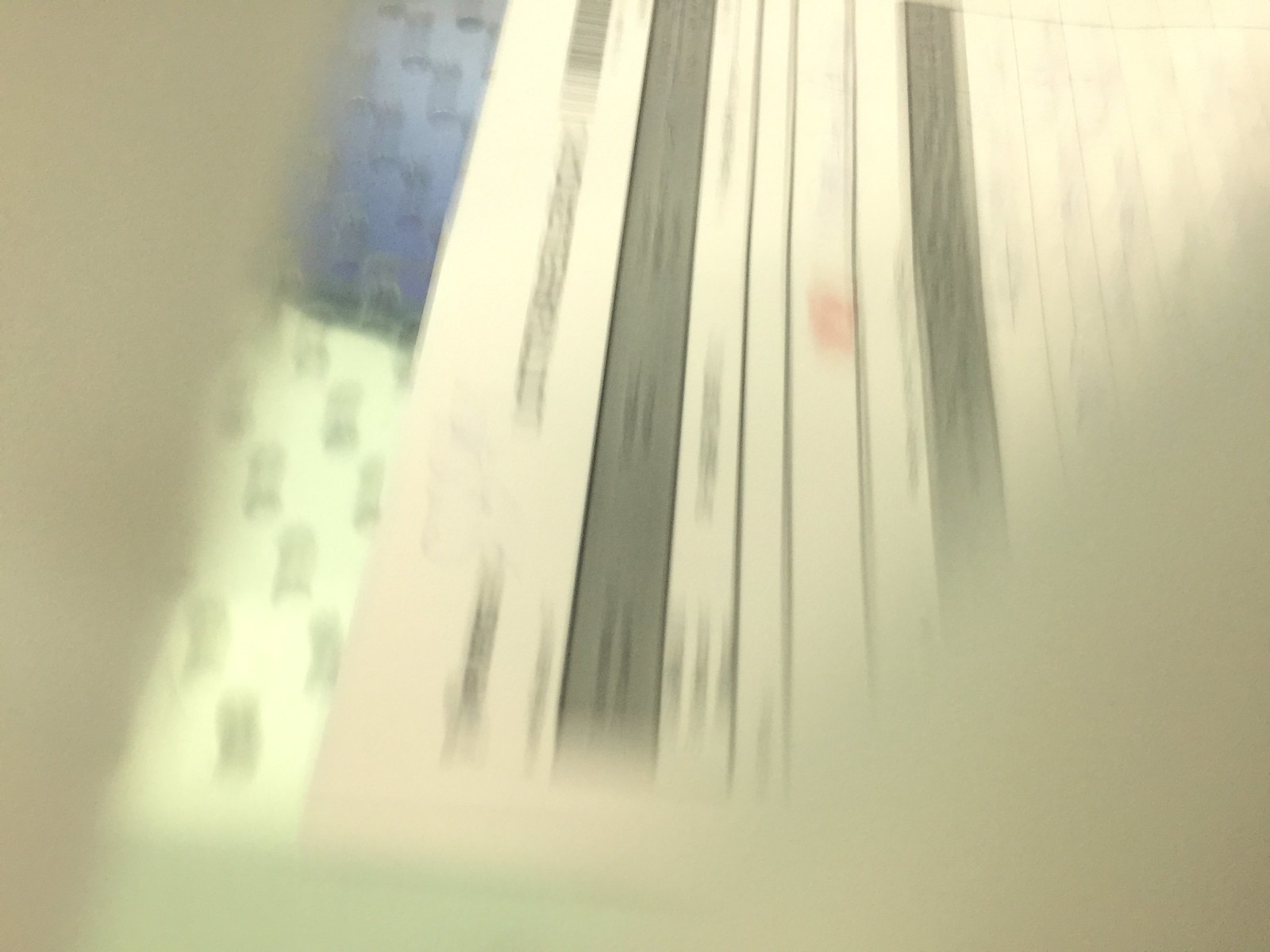This color photograph, though blurred, captures a shelf lined with an assortment of books. On the right side of the image, the photograph is heavily blurred with a pale brownish-gray hue. Above this area, a few white books with their indistinct edges rest on the shelf. Moving leftward, there's a book with a dark border followed by two more paperbacks. All of these appear to be larger paperback editions. Among them, one book stands out with a small red splotch in its center. Continuing left, there are two more white books, a solid gray book, and then a noticeably thicker volume. At the far end, a book features a blue border along the top of its spine that transitions into a white section adorned with numerous green characters. The background color on the far left shifts to a beige-ish brown.